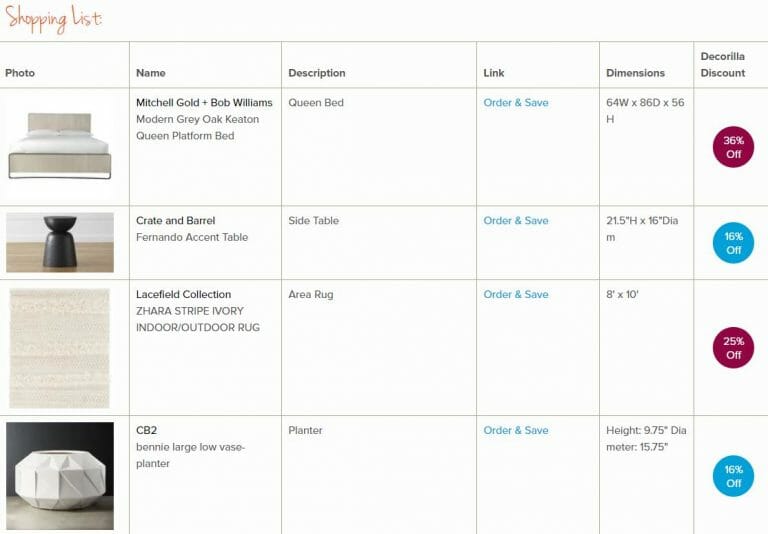**Shopping List**

1. **Item:** Queen Platform Bed
   - **Brand:** Mitchell Gold + Bob Williams
   - **Model:** Modern Gray Oak Keaton
   - **Description:** This stylish queen platform bed features a modern gray oak finish, perfect for contemporary bedrooms. It is available for order and comes with a detailed link for dimensions and additional savings.
   - **Discount:** 36% off

2. **Item:** Side Table
   - **Store:** Crate and Barrel
   - **Description:** A versatile and elegant side table resembling a pottery pedestal, with a chalice-looking top that contrasts with a white base flowing in the opposite direction. Ideal as an accent piece for any living space.
   - **Dimensions:** Provided upon ordering
   - **Discount:** 16% off

3. **Item:** Striped Ivory Area Rug
   - **Brand:** Lanchville Collections
   - **Description:** This beige area rug is adorned with horizontal, multi-colored stripes, adding a subtle yet sophisticated touch to your flooring. It promises to blend seamlessly with various decor styles.
   - **Size:** 8x10
   - **Discount:** 25% off

4. **Item:** Large Low Base Planter
   - **Brand:** CB2
   - **Model:** Benny
   - **Description:** A unique, hexagonal-shaped planter with a modern aesthetic. The geometric cuts add a contemporary flair, making it a striking addition to any indoor or outdoor garden setup.
   - **Discount:** 16% off